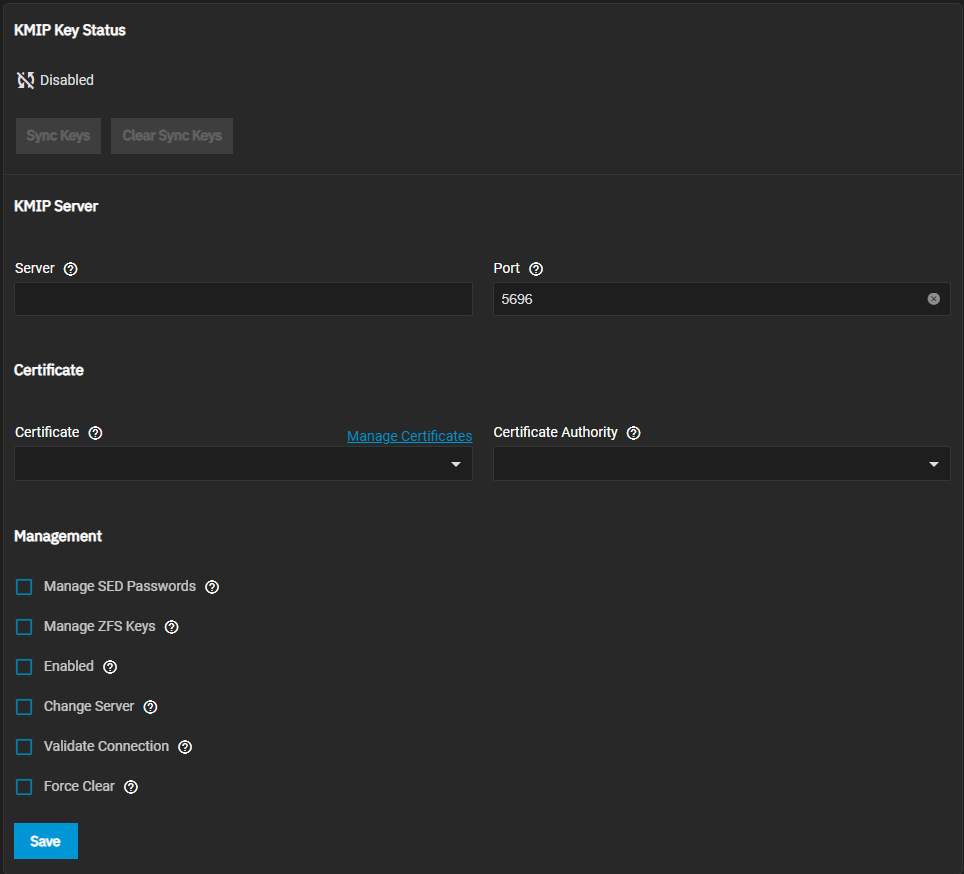This image depicts a KMIP key status page from a KMIP server interface. At the top left-hand corner, the server status is clearly indicated with the term "disabled" in white letters, overlaid with a slash to signify that the server is currently off. 

Moving down, the term "KMIP Server" is prominently displayed alongside a server symbol and the word "Server." Below this section is a black rectangle. To the right, the label "Port" appears in white letters, followed by another black rectangle displaying the number "5696," which likely indicates the port number in use.

Further down, there is an area labeled "Certificate." Within this section, the term "Certificate" is repeated and accompanied by a black rectangle. To the right, a label "Manage Certificates" is displayed with another black rectangle beside it. Above this, "Certificate Authority" is written in white letters.

In the left-hand corner, the page includes a management area with various options, each accompanied by a blue checkbox that can be selected. The options listed are:
- Manage SED Passwords
- Manage ZFS Keys Enabled
- Change Server
- Validate Connection
- Force Clear

Finally, at the very bottom left-hand corner, there is a blue "Save" button for finalizing changes.